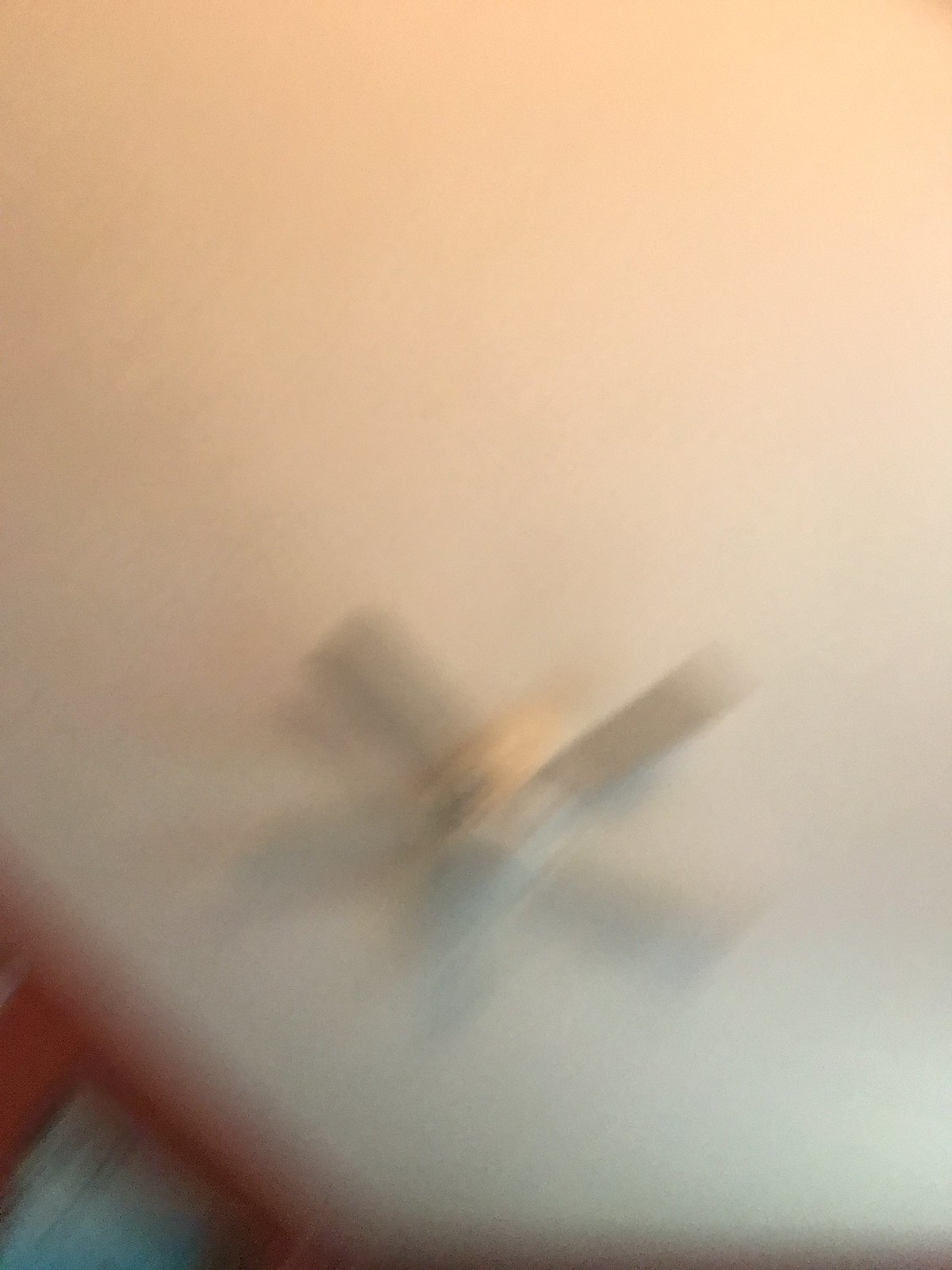The image depicts an extremely blurry photograph of a white ceiling fan with five blades, centered towards the lower part of the frame. The blurriness seems to result from a rapid motion or out-of-focus shot, creating a diagonal motion blur that spans from the top right to the bottom left. The fan is non-operational with visible pull chains. The ceiling fan is set against a white ceiling and is bathed in dim, artificial yellow light, contributing to a grainy, low-quality appearance. The room appears dark and features walls that are painted in a reddish-orange hue. The bottom of the image reveals a small portion of a blue window and some brown wooden trim, adding to the overall muted, natural color palette. There are no people or text in the image, suggesting it was likely taken indoors, possibly from a lying-down perspective on a couch or bed.